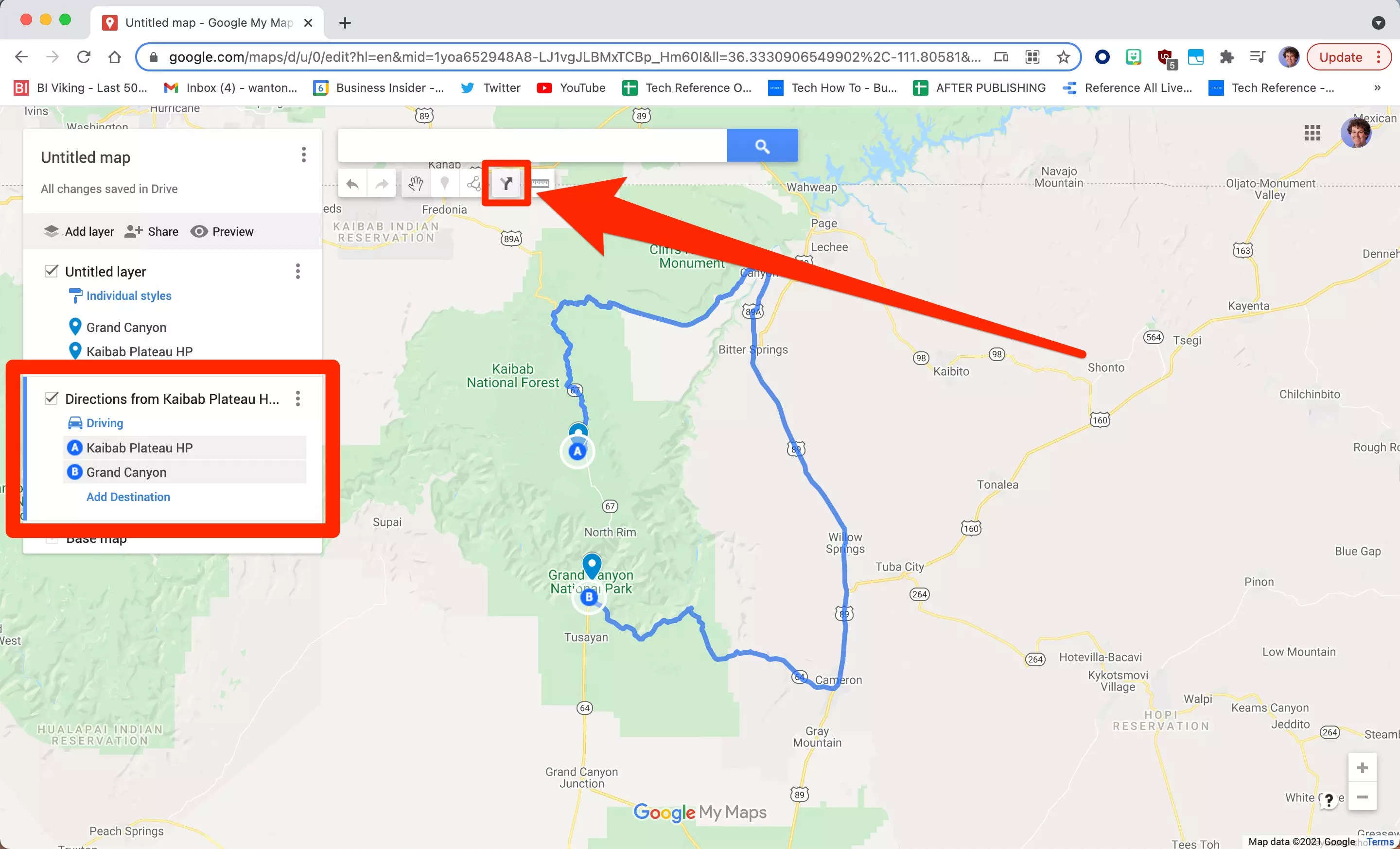This image showcases a web browser window with an active tab displaying a digital map interface. The bookmark bar at the top is populated with various bookmarks including "Viking Last 50," "Inbox 4," "Wanton," "Business Insider," "Twitter," "YouTube," "Tech Reference," "Tech How-To," "After Reference All Live," and another "Tech Reference" bookmark. 

On the left side of the screen, the map interface panel lists details such as "Untitled Map," "All Changes Saved," and options including "Drive," "Add Layer," "Share," "Preview," and "Untitled Layer." Further down, there are text labels for "Individual Styles," "Grand Canyon," "K-Bob Plateau," a checkbox labeled "Direction from K-Bob Plateau Driving," followed by mentions of "K-Bob Plateau," "HP," and "Grand Canyon." A blue hyperlink reads "Add Destination."

The entire map interface section is outlined in red, and a red arrow is pointing to an icon situated below the search bar. This icon is likely related to navigating or managing the displayed map.